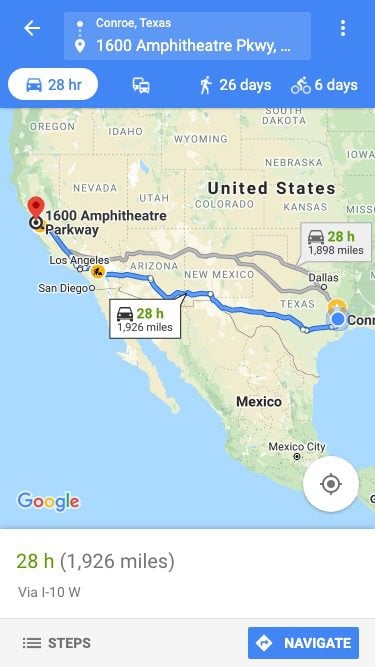A detailed caption for this image could be:

This is a detailed screenshot of a Google Maps navigation page. At the top, the current location is listed as Conroe, Texas, with the destination set to 1600 Amphitheater Parkway, followed by ellipses. Just below this header, the estimated travel time is displayed as 28 hours alongside a car icon that is highlighted, indicating the selected mode of transportation. To the right of this, alternative travel modes and their respective times for bus, walking, and biking are presented.

Dominating the screen is a map view that spans a large portion of the United States, stretching from South Texas to California. A prominent blue line represents the main driving route, accompanied by two alternate routes depicted in gray. Centered along the primary route is a white pop-up box indicating a travel time of '28 H' in green, with a car icon to its left and a distance of 1,926 miles below.

The bottom left corner features the Google logo, while the bottom right displays a white circle with a location icon.